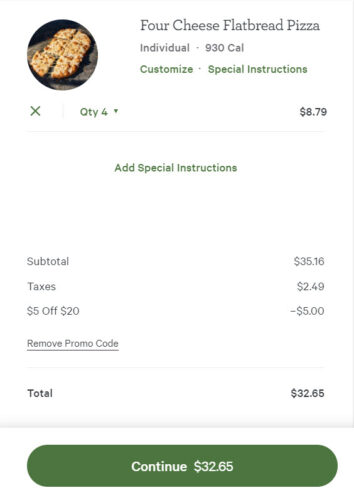**Order Summary: Four Cheese Flatbread Pizza**

This screenshot, captured from a mobile application, shows a detailed view of an order placed online. The image exhibits a clean, white background.

- **Top Left Corner:** A circular thumbnail image of the product.
- **Product Title:** "Four Cheese Flatbread Pizza" positioned to the right of the thumbnail.
  - **Description:** Listed as "Individual" with a calorie count of 930.
  
Underneath the product title:
- **Customize Button:** An option to add special instructions.
- **Quantity and Pricing:** Displayed prominently as four pizzas at $8.79 each.
  - **Subtotal:** $35.16
  - **Taxes:** $2.49
  - **Coupon Applied:** A $5 discount for orders over $20.
  
The final total for the order is $32.65, after applying the coupon and including taxes.